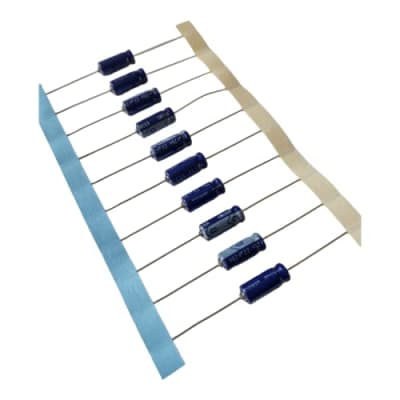This detailed, close-up photo showcases a meticulously organized row of resistors, each aligned horizontally and parallel to one another, creating a pattern reminiscent of a ladder. The resistors are evenly spaced along a strip of tape, with the left side featuring blue painter's tape and the right side white painter's tape. Each resistor has silver leads extending from a central dark blue cylindrical body adorned with a light blue stripe. The resistors are uniformly laid out across the white background, starting diagonally from the upper left to the lower right corner of the image. The background is entirely blank, drawing full attention to the uniformly spaced resistors, which appear to have just been unpackaged and are ready for use. This image likely serves a purpose in advertising or a marketplace, highlighting the neat arrangement and high-quality appearance of the resistors.